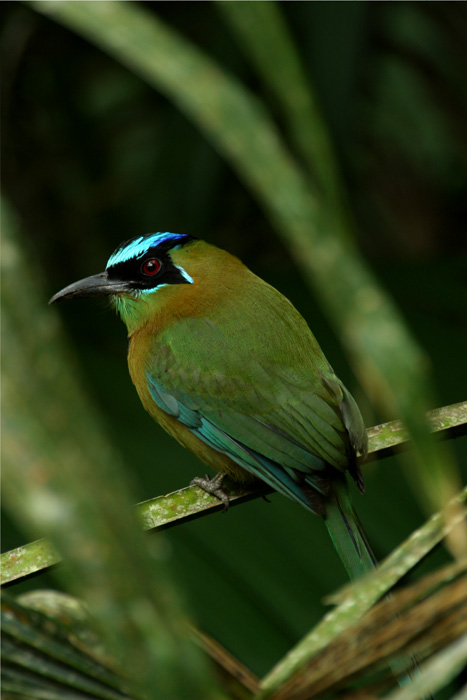A close-up portrait photograph captures a small, textured green bird perched on a structurally sound, long green leaf, likely from a palm tree. The background is softly blurred in varying shades of dark green, light green, and black, emphasizing the bird's vivid details. The bird is predominantly green, with shades transitioning to light green and tannish gold yellow along its body. Strikingly colorful, it features brilliant neon blue accents on its crown and underneath its eyes, contrasting with its black face which has a mask-like appearance around its distinctive reddish-brown eyes. The bird's beak is slender and pointed, a grayish hue. The scene is complemented by other similar leaves, adding to the natural ambiance.